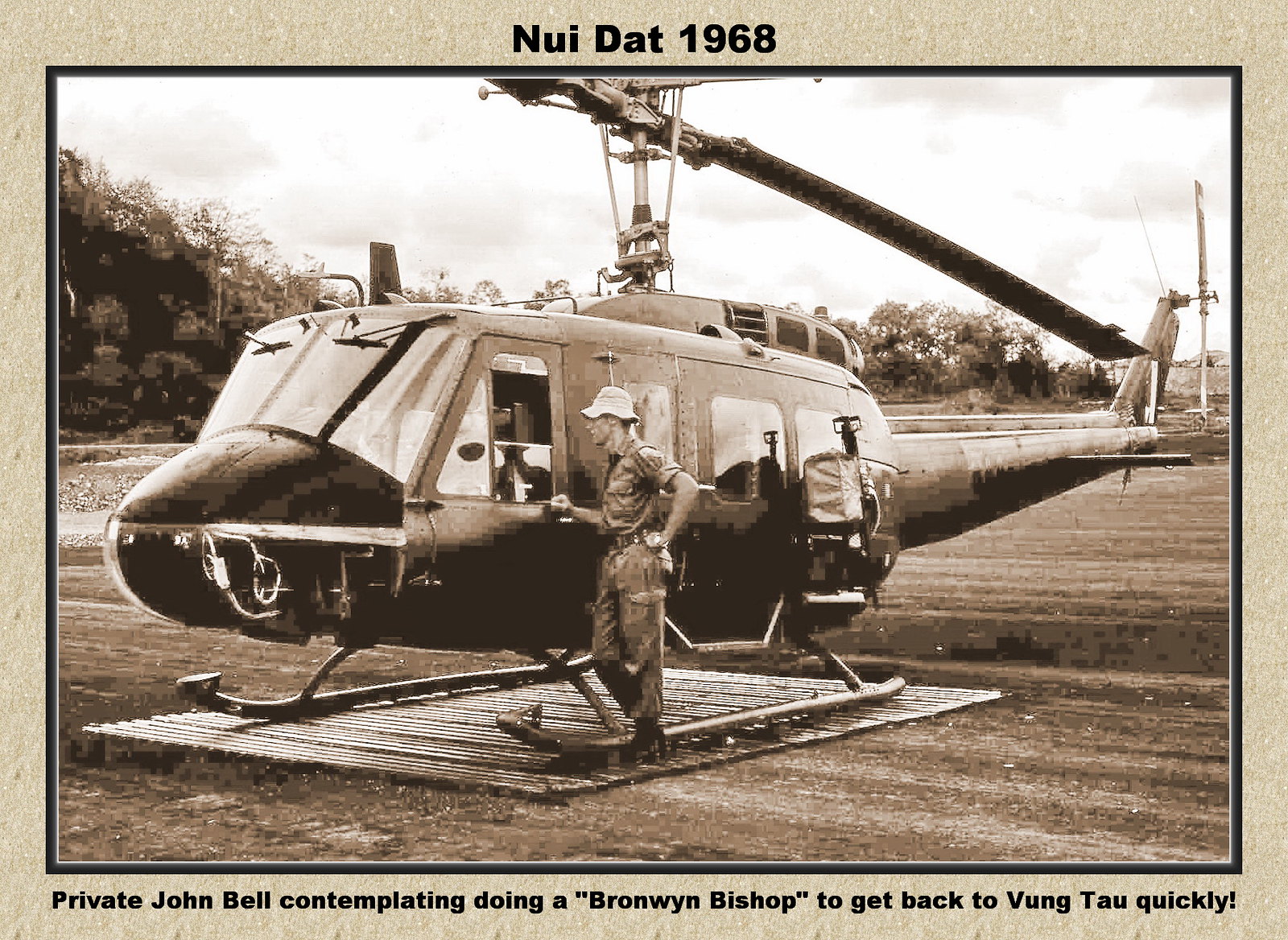The image is a card from the Vietnam War era, framed by a light tan or gray recycled paper-like border. At the top, it reads "Nui Dat, 1968," while the bottom text states, "Private John Bell contemplating doing a 'Bronwyn Bishop' to get back to Vung Tau quickly!" The center photo, bordered in black and dark brown, is a sepia-toned, brown-and-white photo showing a soldier in army fatigues standing on a makeshift square wooden landing pad. He is facing and looking into the front side window of a helicopter, perhaps speaking to the unseen pilot. The helicopter is stationary, with its rotors still, suggesting an idle moment in a war zone. The background depicts a barren field with sparse grass or dirt, possibly reflecting winter conditions, and a line of trees under a cloudy sky, adding to the somber and timeless feel of the scene.